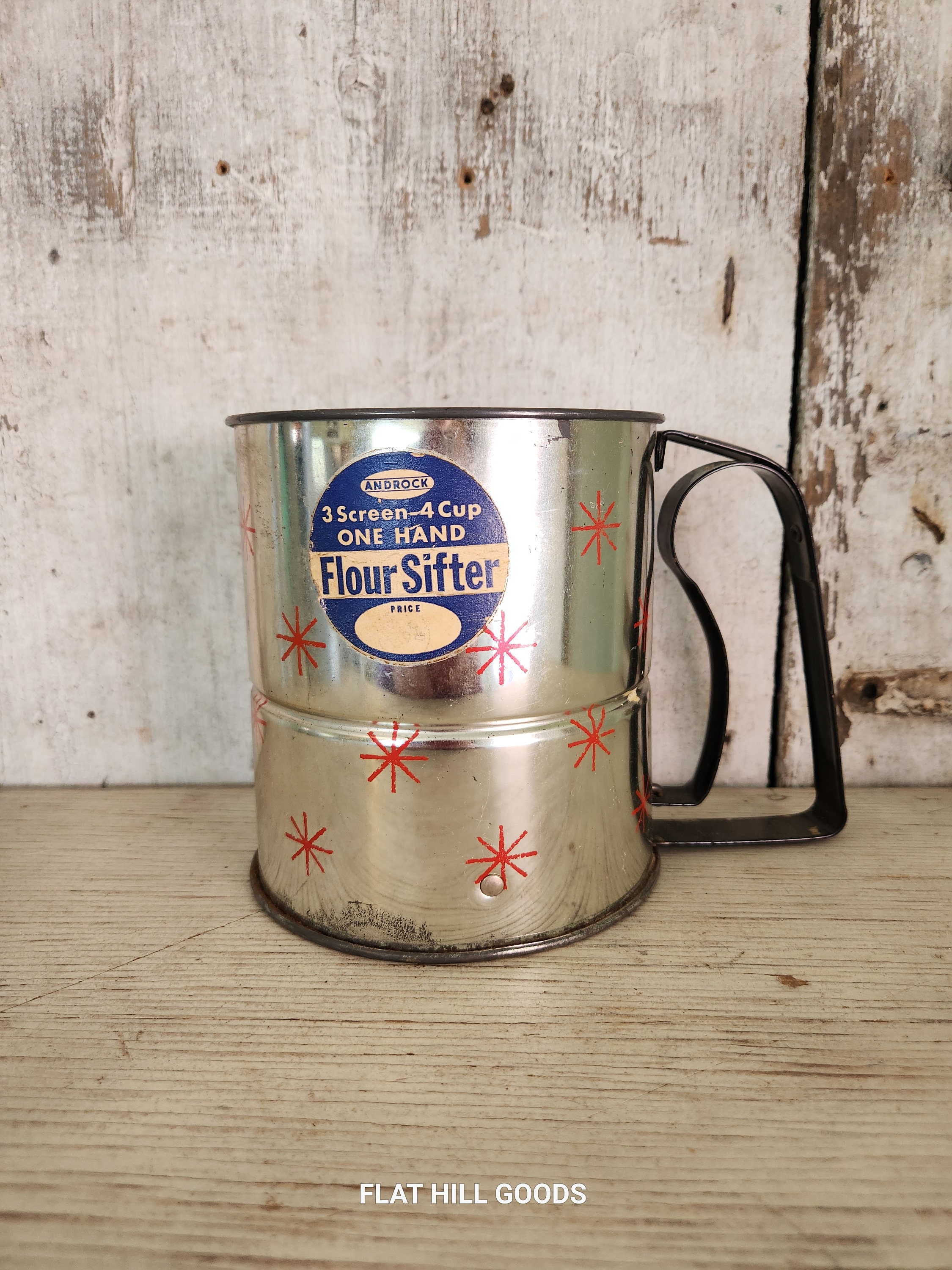The photograph features a rustic scene with an antique flour sifter as the central focus. The sifter, a silver cylindrical metal device with a black handle on the right side, is adorned with red asterisks that form a star-like pattern. A blue and white circular sticker on the top front of the sifter reads, "Androck three screen, four cup, one hand flour sifter." The sifter rests on a wooden tabletop or shelf that occupies the lower 40% of the image, painted off-white with sections of worn, brown wood showing through. Behind the sifter, the background comprises two large wooden planks, similarly painted white and worn, revealing the original wood underneath. The backdrop also features a few nail holes, adding to the rustic charm. Across the bottom of the image, in the center, white text reads, "Flat Hill Goods."